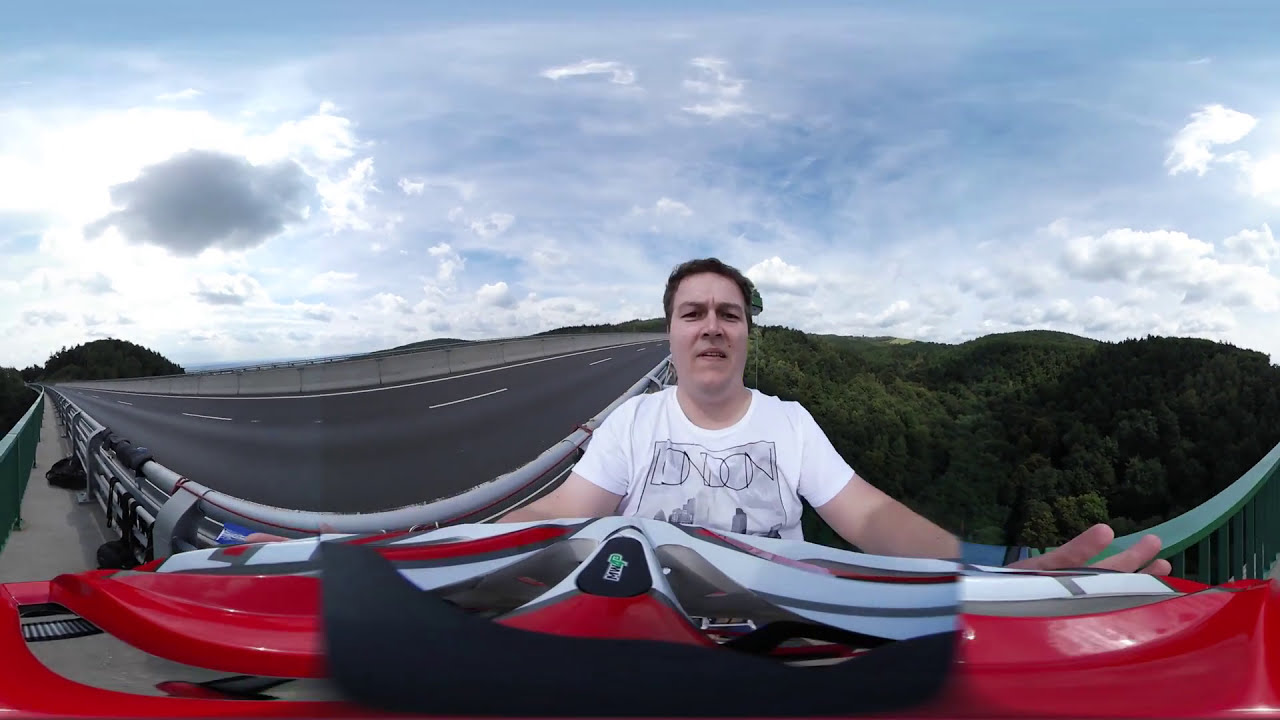A young person with short brown hair is taking a selfie, likely with the help of a selfie stick, while standing on a bridge. They're wearing a white t-shirt with the word "London" printed on it. In their hands, they're holding a large, glossy red object that seems to be part of a motorcycle, possibly a mud flap or handlebar, though it might also resemble a drone. The image has some distortion due to filter effects and appears to be stitched from multiple 360-degree camera shots, resulting in a slightly warped view. Behind the person is a paved, single-lane road that curves to the right, flanked by green steel guardrails. The bridge overlooks a lush valley filled with dense green trees. The sky above is a mix of blue with lots of gray and white clouds, some appearing heavy with moisture, casting a muted light on the scene. The person appears to be on the pedestrian walkway of the bridge, near a bungee harness and mounting point attached to the guardrail.